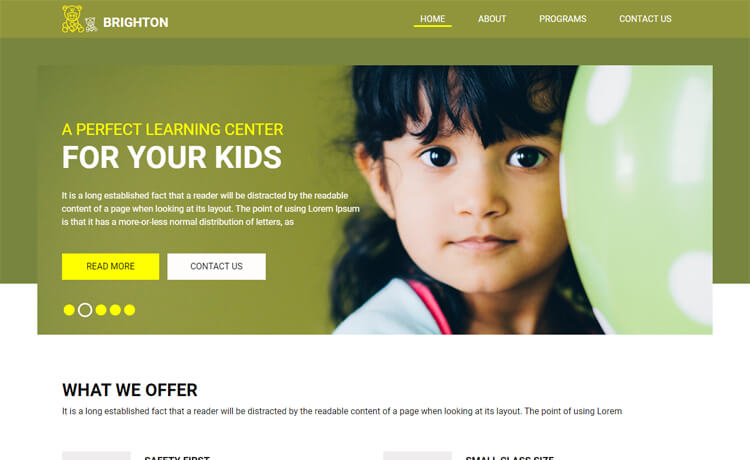This image depicts a webpage for a learning center in Brighton, characterized by a coherent design and clear labeling. At the top left corner, there's an icon featuring a yellow outline of a teddy bear, juxtaposed against a white background with the "Brighton" text prominently displayed. The navigation menu is aligned to the right, featuring options for "Home," "About," "Programs," and "Contact Us" in uppercase white text, with the "Home" section underlined in yellow, indicating the current page.

The overall background has an olive green hue, creating a soothing and professional atmosphere. Below the navigation bar, the main background shifts to a darker slate or olive green color. Dominating the central part of the webpage is an outlined image box with a yellow border on the left side. A headline within this section reads "A Perfect Learning Center" in all caps. Beneath this, larger white text adds, "For Your Kids," providing a welcoming message to visitors.

Further down, there is placeholder text: "It is a long established fact that a reader will be distracted by the readable content of a page when looking at its layout. The point of using Lorem Ipsum is that it has a more-or-less normal distribution of letters." This is accompanied by call-to-action buttons labeled "Read More" and "Contact Us."

On the right side of the central section, there's an image of a young girl with black hair, who appears to be of Indian descent. The girl is closely accompanied by a light green balloon with white polka dots, adding a playful and inviting element to the webpage. The design elements and color palette combine to create a vibrant yet educational ambiance, suitable for a learning center's online presence.